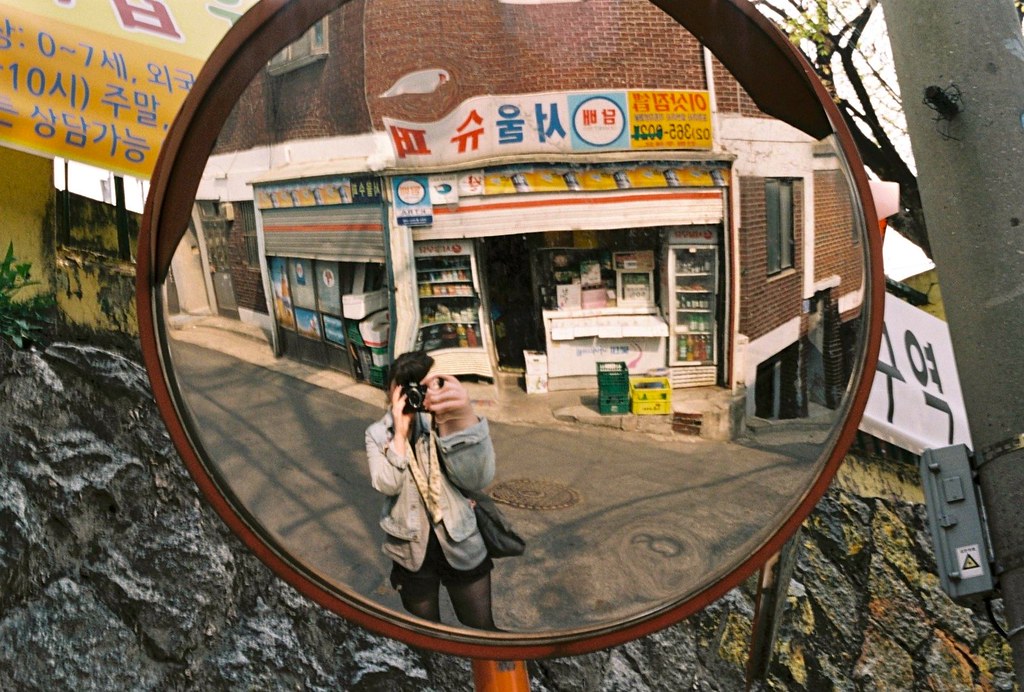The image depicts a person with a black camera obscuring their face, standing outside in front of what appears to be a market. The person is wearing black shorts, nylons, and a jean jacket, or possibly a gray suit jacket. They are taking a photo reflected in a large, circular mirror, creating a somewhat surreal effect. The person's left hand appears distorted and much larger than the right, likely due to the mirror's curvature. The market behind them has signage with Asian lettering—possibly Chinese or Korean, with characters in red and blue—that labels the storefront. The building is constructed from red and light brown bricks, and it is situated on a street corner with green and yellow newspaper stands or boxes visible outside. The overall composition gives a trippy, reflective feel with the market's details and the person's distorted reflection standing out prominently.